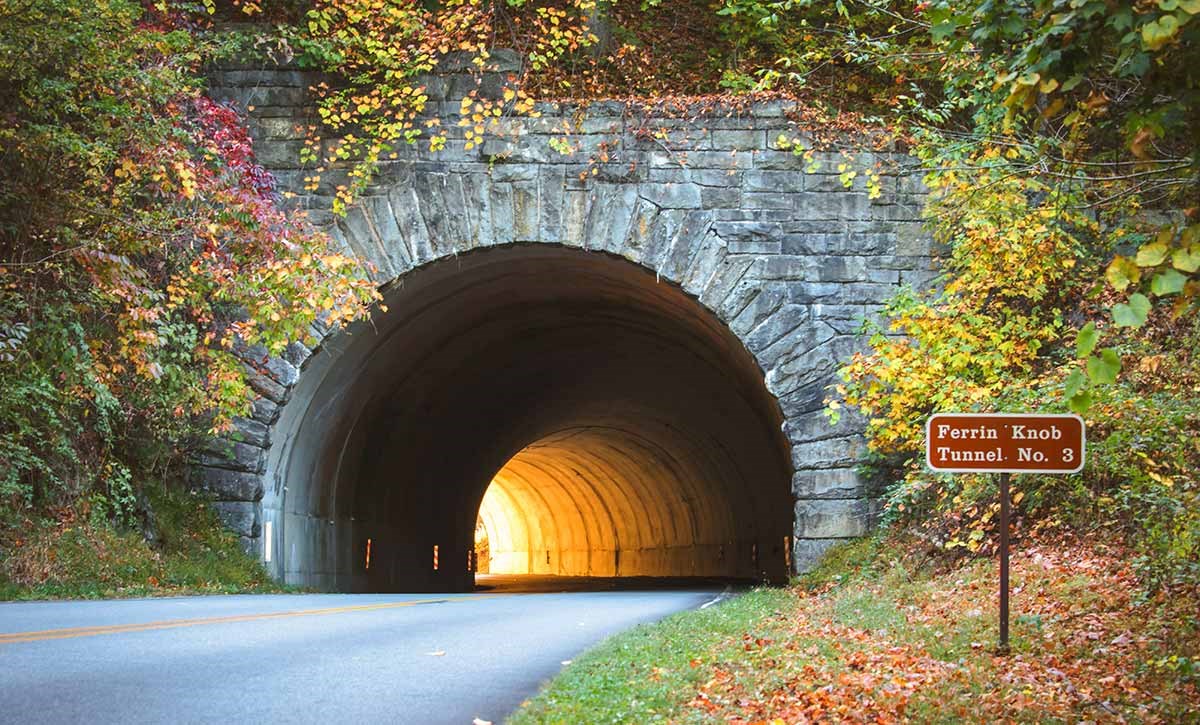In this detailed photograph, a winding roadway leads directly toward the Farran Knob Tunnel Number 3, an arched passage carved into the side of a stone hill. The tunnel, constructed from sturdy gray stone interspersed with dark grays, light grays, and hints of rust, exudes a rugged and weathered charm. Surrounding the tunnel entrance, lush foliage, including various trees and bushes, drape over the stone, with some of the vegetation beginning to show the vibrant colors of autumn—reds, oranges, and browns. This seasonal change is evidenced by the fallen leaves scattered around the entrance and the leaves turning colors among the overgrowth. The top portion of the tunnel structure is nearly obscured by this lush greenery. A brown sign with a white border stands prominently near the entrance, clearly reading "Farran Knob Tunnel Number 3." The tunnel appears well-lit from the far end, presumably by sunlight, signalling that it is relatively short and curved to the left, disappearing from direct sight. A patch of grass is visible on the right-hand side, enhancing the natural surroundings of this picturesque scene.